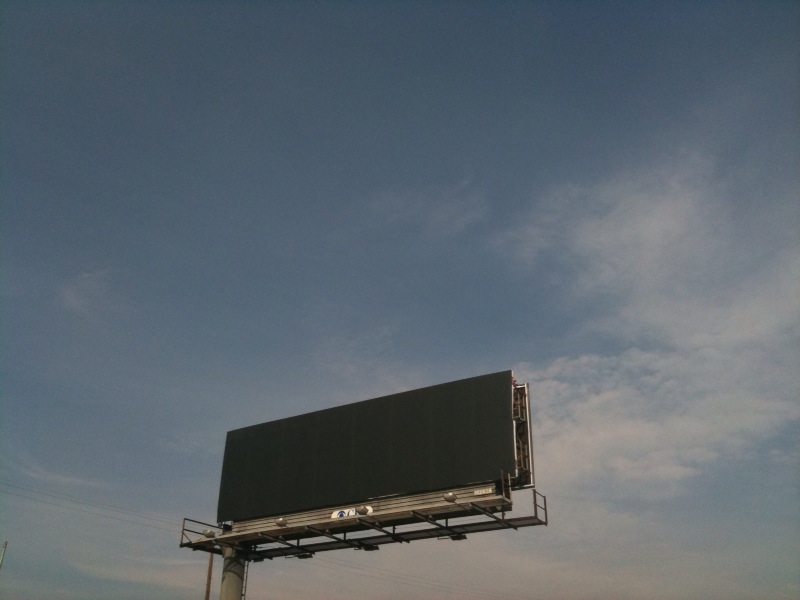The photograph captures a large, double-sided, empty billboard perched atop a towering steel structure. The billboard, a black rectangle devoid of any advertisements, stands prominently against a dramatic dusk sky. The sky transitions from a darker blue at the top left to lighter hues infused with pink on the right, adorned with wispy white clouds. The sturdy, dark gray pillar supporting the sign is positioned on the left, casting a shadow at its top. The billboard's framework features light gray and dark gray scaffolding, designed for maintenance purposes. Silver light housings jut out from the billboard, although they remain unlit, suggesting it is still midday or early evening. A white plaque with numbers is affixed at the bottom of the structure. Overall, the scene evokes a calm yet striking impression of an industrial installation against a picturesque twilight sky.